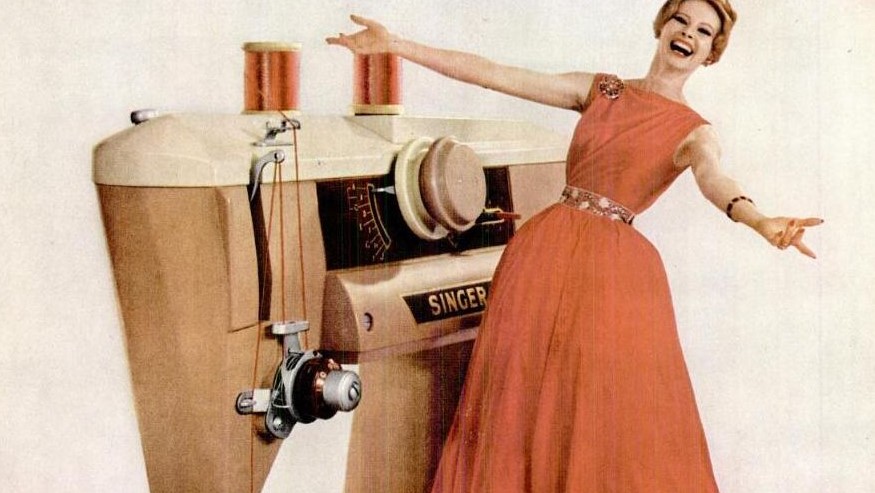In this vintage advertisement, a cheerful woman stands beside an oversized Singer sewing machine. Dressed in a sleeveless, orange-red dress adorned with a golden, possibly gold and red belt or waistband, she extends her arms wide open, her body slightly leaning back, radiating joy with a big smile that reveals the top row of her teeth. Her hair is styled in tight curls close to her scalp, and she accessorizes with a bracelet and a prominent brooch on her left shoulder. The Singer sewing machine, nearly as tall as the woman, is a striking combination of brown and cream with various knobs and sewing instruments, supporting two peach-colored spools of thread on top. The background is a simple light grey, which helps to highlight the vivid colors and details of both the woman and the machine. The machine's brand name, 'Singer,' is clearly visible, enhancing the vintage, advertisement-like feel of the image.